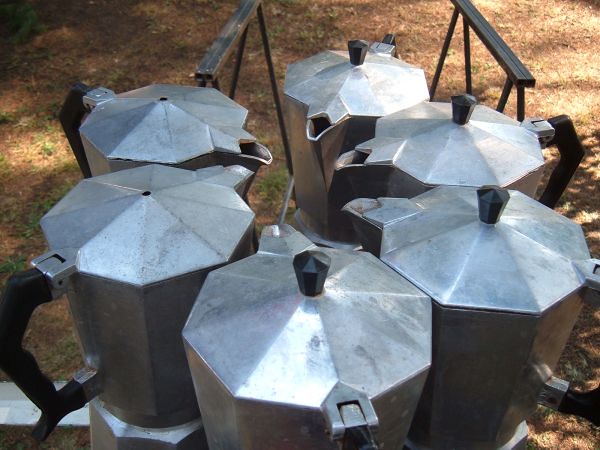This image captures six vintage, stainless steel coffee pots arranged in a circle with their spouts facing inward towards the center, creating a symmetrical ring-like formation. Viewed from above, these pots display shiny silver tops and dark gray outer bases. Notably, four of the pots have small knobs on their hexagonal-shaped lids, while two are missing these features. Each pot has a black handle that appears softer and contrasts with the metal body. The scene is set outdoors under the shade, with a barrier visible in the background. The ground beneath the pots is predominantly brown, interspersed with patches of green grass, possibly suggesting they're placed on a step or patio area.